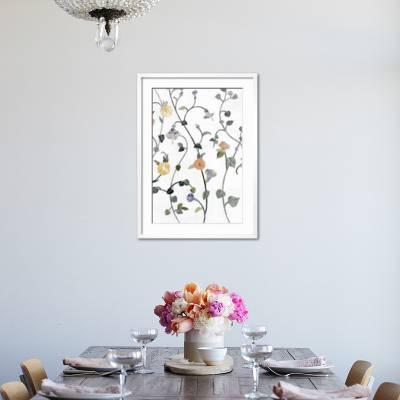This photograph captures a detailed view of a dining room. The room is illuminated with a hint of blue, set against an off-white or subtly blue-tinged background. At the top of the image, slightly offset to the left, a clear or crystal light fixture with a black attachment can be seen hanging from the ceiling. Centrally positioned on the wall is a white-framed painting depicting a delicate vine plant adorned with small flowers, resembling baby's breath, enhancing the simplicity and elegance of the setting.

Below this artwork is a prominently featured wooden dining table, dark brown in color, accompanied by four chairs, the tops of which have a yellow hue. The table is meticulously set for four, each place setting comprising a plate, silverware wrapped in a napkin, and a wine glass. In the center of the table, a white pot filled with an arrangement of pink, white, and yellow flowers adds a vibrant touch to the scene. Additionally, a teacup is placed in front of the floral centerpiece, completing the charming dining setup. This comprehensive view encapsulates the essence of a fashionably arranged dining room, blending functionality with aesthetic appeal.